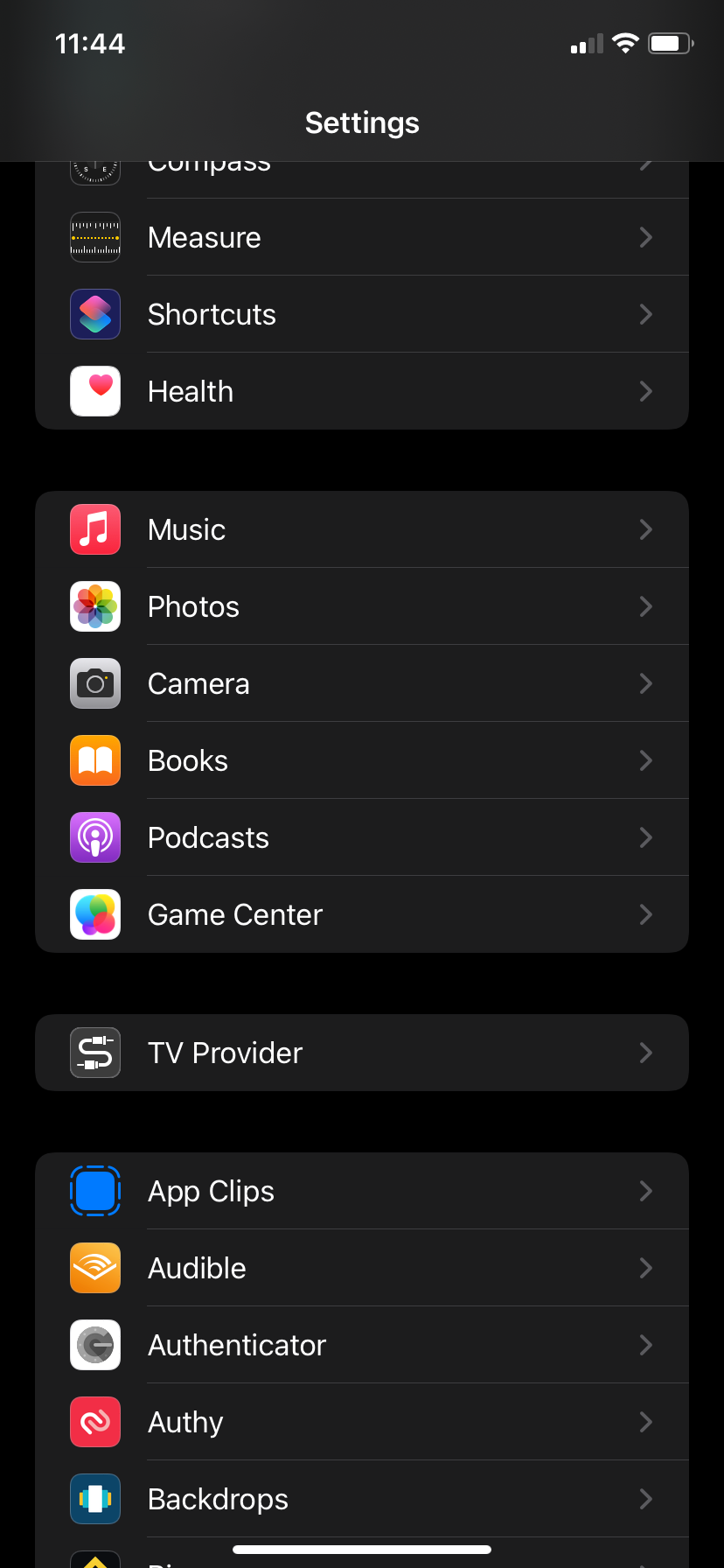This image captures the screen of an Apple device displaying its Settings menu. The screen appears to be partially scrolled down, showcasing a variety of settings and app sections. At the very top visible section, there are grouped settings for Compass, Measure, Shortcuts, and Health, indicating other sections are likely hidden above due to scrolling. Following this group, there is another set that includes Music, Photos, Camera, Books, Podcasts, and Game Center. Below this, the TV Provider option is listed independently. Further down, there is a grouping of third-party apps including App Clips, Audible, Authenticator, Authy, and Backdrops. Each setting is accompanied by a corresponding icon on the left and a right-pointing arrowhead on the right, indicating further options within each section.